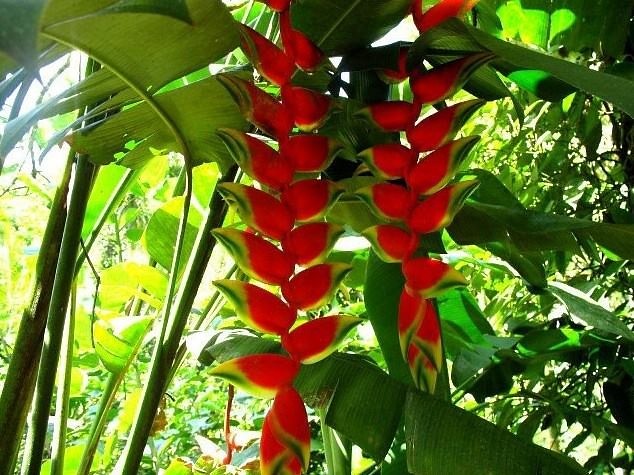In this captivating outdoor scene, we find ourselves peering through dense jungle vegetation, where the sunlight barely pierces the thick foliage above, highlighting the scene predominantly on the left side with its radiant glow. Surrounded by an abundance of large, frond-like leaves that dominate the background, our view is partially obscured by this lush greenery. 

In the foreground, two distinct plants draw immediate attention. Rising from the bottom to the top of the image, these plants feature stalks adorned with alternating petals arranged like a zipper. These petals, light red in color, cascade down each stalk in a striking pattern. Each stalk is laden with what appears to be teardrop-shaped fruits or flowers, forming delicate chains. These red teardrops, numbering about a dozen on each stalk, dangle in double rows, creating a vivid contrast against the sea of green leaves. The entire scene evokes the essence of a jungle or a rich garden brimming with life and color.